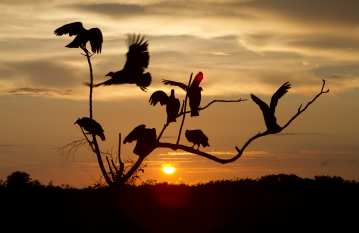The image captures the serene beauty of a sunset, with the sky painted in a mesmerizing combination of oranges, pinks, and blues. In the foreground stands a tree with several bare branches—one extending upward, while others curve to the right. The tree, without any visible leaves, serves as a perch for eight birds, silhouetted against the vibrant sky. Some birds sit closely together, their shapes dark against the colorful backdrop, with one bird noticeably taking flight to the left. Below the tree is a patch of dark, indistinct plant matter, likely grass, not clearly visible due to the low lighting. On the horizon, a ball of the setting sun casts its brilliant glow, while the distant outline of a forest appears in shadow. High above, clouds reflect the warm hues of the sunset, completing this tranquil scene.